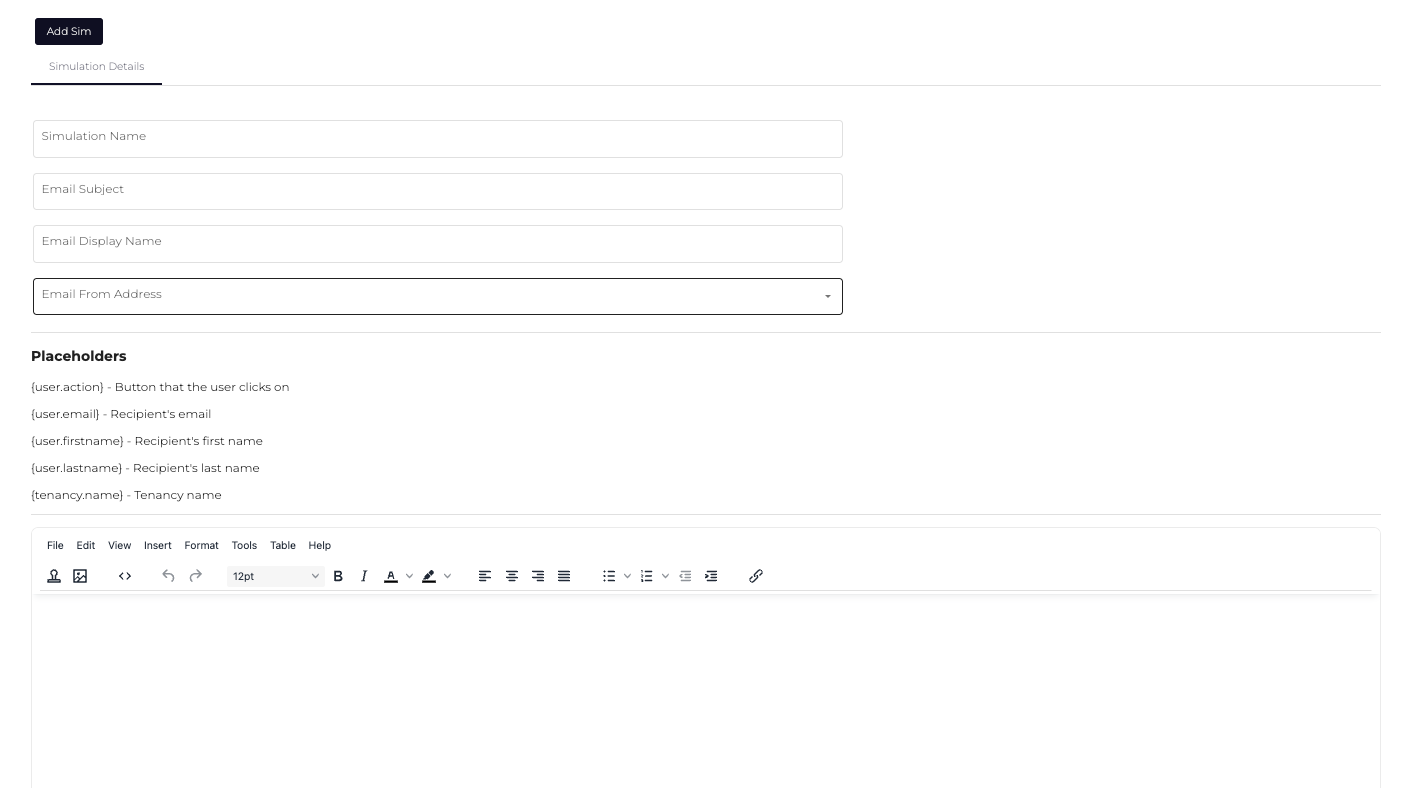The image showcases a user interface of a form with low resolution, making some text difficult to read. The top left corner features a black button labeled "Add SIM." Directly beneath, a section titled "Simulation Details" is underlined, containing several fields with default text. The first field reads "Simulation Name," followed by "Email Subject," "Email Display Name," and "Email From Address." The last field has a darker border, emphasizing its importance.

Below these fields, a gray line demarcates the beginning of a section titled "Placeholders," highlighted in dark, bold text. Listed placeholders include:
- "user.action" / "user.action.button" (the button the user clicks on)
- "user.email" (recipient's email)
- "user.firstName" (recipient's first name)
- "user.lastName" (recipient's last name)
- "tenancy.name" (tenancy name)

Further down, another line is followed by a horizontal row of buttons labeled "File," "Edit," "View," "Insert," "Format," "Tools," "Table," and "Help," resembling a typical Notepad-like interface.